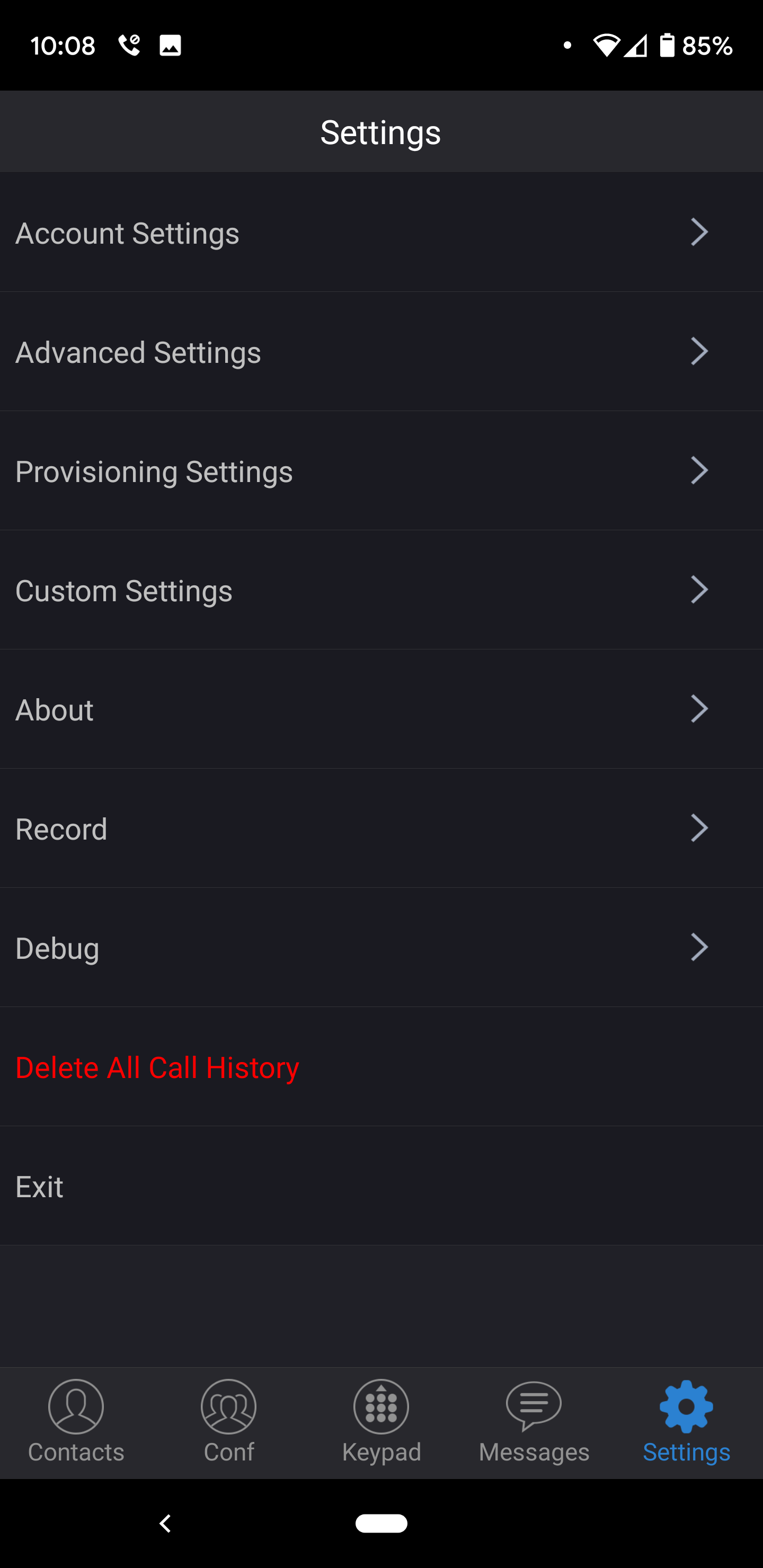This image is a detailed screenshot of a settings page on a mobile device. Across the top, there's a dark grey bar with the word "Settings" prominently displayed in white text at the center. 

Immediately below this header, there are seven distinct options organized in a list, each with descriptive text on the left and a forward arrow icon on the right, indicating further navigation. The options are as follows: "Account Settings," "Advanced Settings," "Provisioning Settings," "Custom Settings," "About," "Record," and "Debug."

Beneath these seven buttons, there is a distinctive red button labeled "Delete All Call History." Following this is a light grey "Exit" button.

At the very bottom of the screen, there is another grey bar containing five navigation buttons, each accompanied by an icon located above the respective text. These buttons are labeled: "Contacts" (represented by a contacts icon), "Conf" (likely short for conference, with an appropriate icon), "Configuration" (with a relevant icon), "Keypad" (accompanied by a keypad icon), and "Messages" (illustrated with a messages icon). The gear icon, symbolizing settings, is highlighted in blue.